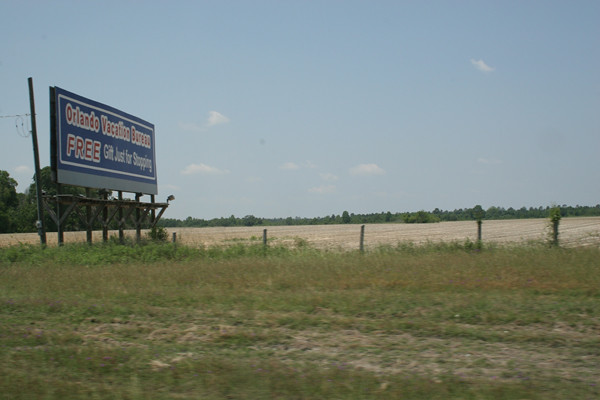This digital photograph, though of lower quality, captures a tranquil rural scene presumably near Orlando. Viewed from the side of the road, the image reveals a flat, expansive field showing signs of drought, with yellowish-gray hues dominating the landscape under a pale blue sky. In the foreground, a gentle, grassy bank, interspersed with patches of dirt, leads up to the field. On the left side of the photograph stands a modest, slightly weathered billboard that reads "Orlando Vacation Bureau - Free Gift Just for Shopping." A series of fence posts lines the edge of the bank, demarcating the boundary between the grassy verge and the dry field beyond.